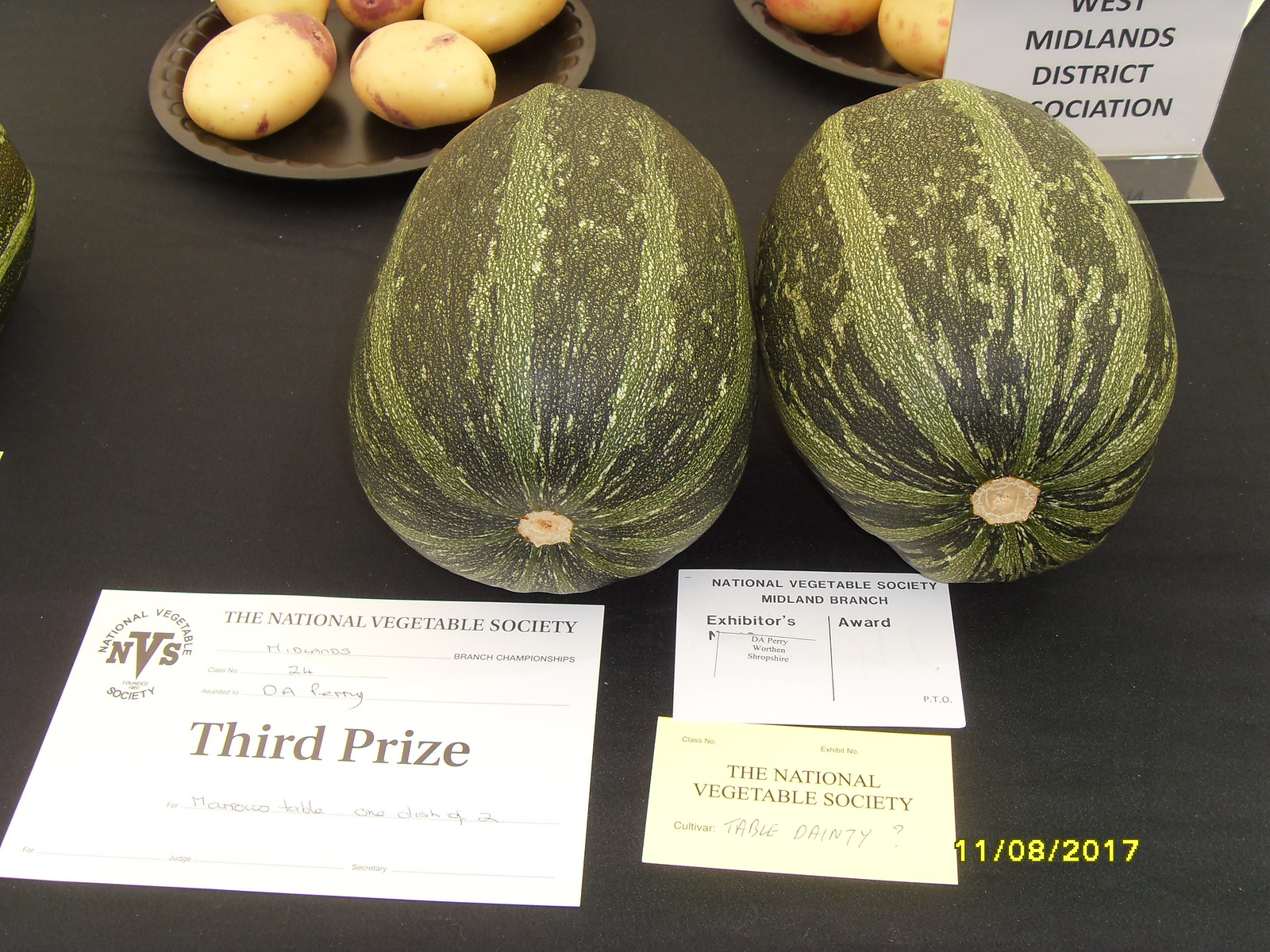The image displays a selection of green watermelons arranged on a black tablecloth, taken at a vegetable competition dated 11-08-2017. On the left-hand side of the frame, bowls containing peeled white potatoes rest next to a brown plate with more potatoes, both featuring the label "West Midlands District Association." The display also includes several awards and informational cards: a white document from the National Vegetable Society outlining third-prize details, another card bearing the National Vegetable Society Midland Branch Exhibitors Award title, and a business-type card. The National Vegetable Society's logo and related details are visible on various plaques and sheets throughout the setup.